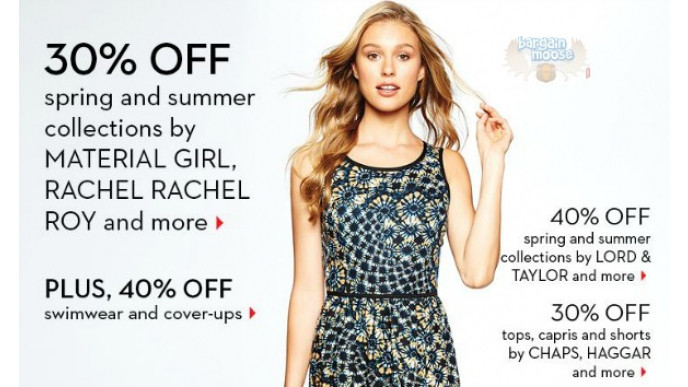This digital advertisement features a light gray background with prominent promotional text and an image of a fashionable woman. 

In the top left corner, large black text announces "30% OFF." Directly below, slightly smaller text reads "SPRING AND SUMMER COLLECTIONS BUY." Following this, in all caps, the brands "MATERIAL GIRL" and "RACHEL RACHEL ROY" are listed, along with "and more" in smaller lowercase text. A red arrow points to the right, indicating further information.

Further down, separated by some negative space, bolded black text states "PLUS 40% OFF," with smaller text beneath it saying "SWIMWEAR AND COVERUPS," accompanied by another red arrow pointing to the right.

In the center of the image, a blonde woman poses in a sleeveless dress adorned with a peacock tail feather print. She holds a lock of her hair up with her left hand. 

In the top right corner, there is a watermark featuring a logo with cartoon moose antlers mounted on a plate. Above the logo, in blue outlined cartoon-style text, it says "BARGAIN MOOSE," with a red sale tag hanging from the antlers.

In the bottom right section, two paragraphs of black text provide additional offers. The first paragraph reads "40% OFF, SPRING AND SUMMER COLLECTIONS BUY, LORD AND TAYLOR," highlighted in all caps, followed by "and more" and a red arrow pointing to the right. Below this, another paragraph states "30% OFF," and in lowercase text, details "TOPS, CAPRIS, AND SHORTS BUY," followed by "CHAPS, HAGGAR" in uppercase, and "and more" in lowercase, with a red arrow pointing to the right. Both "40% OFF" and "30% OFF" are slightly larger and in caps but are not bolded.